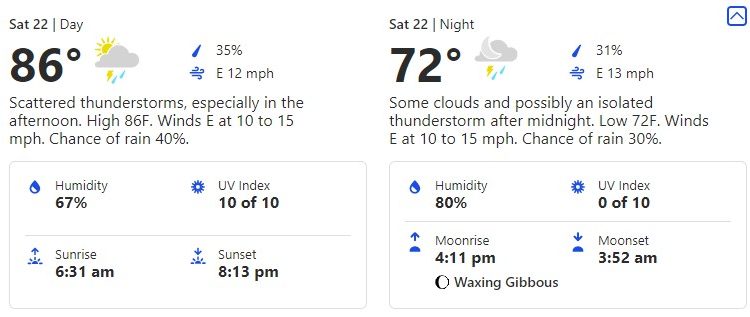**Descriptive Weather Forecast for Saturday, 22nd**

**Daytime Forecast:**
- **Temperature:** 86°F
- **Weather Icon:** Partly cloudy with scattered thunderstorms depicted by a gray cloud with the sun peeking behind it, a yellow lightning bolt, and blue raindrops.
- **Rain Probability:** 35% (shown to the right of the icon with a raindrop)
- **Wind:** East at 12 mph (represented by a logo "E 12mph")
- **Detailed Forecast:** Scattered thunderstorms, especially in the afternoon. High of 86°F. Winds east at 10 to 15 mph. Chance of rain is 40%.
- **Additional Details:**
  - **Humidity:** 67% (indicated by a water droplet half filled with blue)
  - **UV Index:** 10 out of 10 (shown with a blue sunshine icon)
  - **Sunrise:** 6:31 AM (depicted by a sun with an upward arrow)
  - **Sunset:** 8:13 PM (illustrated with a sun and a downward arrow)

**Nighttime Forecast:**
- **Temperature:** 72°F
- **Weather Icon:** Cloudy with a possible isolated thunderstorm depicted by a gray cloud with a moon, a yellow lightning bolt, and blue raindrops.
- **Rain Probability:** 31% (presented to the right of the icon with a raindrop)
- **Wind:** East at 13 mph (indicated by the same logo "E 13mph")
- **Detailed Forecast:** Some clouds with a possibility of an isolated thunderstorm after midnight. Low of 72°F. Winds east at 10 to 15 mph. Chance of rain is 30%.
- **Additional Details:**
  - **Humidity:** 80% (shown with a water droplet half filled with blue)
  - **UV Index:** 0 out of 10 (displayed with a blue sunshine icon)
  - **Moonrise:** 4:11 PM (illustrated by a moon with an upward arrow)
  - **Special Note:** Waxing Gibbous phase (depicted by a circle with a tiny black edge colored in)
  - **Moonset:** 3:52 AM (represented by a moon with a downward arrow)